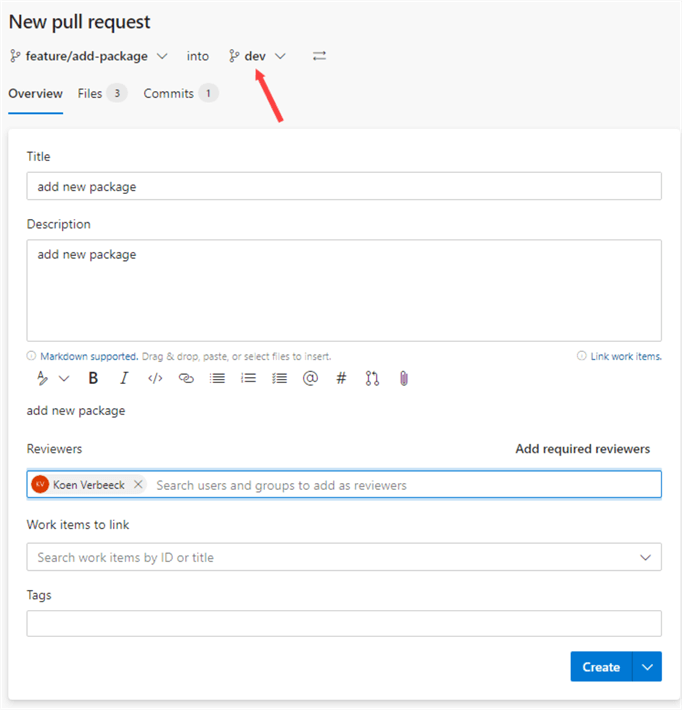The image displays a user interface for creating a new pull request. The top section has a gray background, and on the left-hand side, the text "New Pull Request" is prominently displayed in black font with a capital 'N'. Below this, it reads "feature/add-package", indicating the feature branch. An arrow points downward, leading to the text "into DEV", suggesting the target branch for the merge, accompanied by a mysterious red arrow pointing down.

On the next row, the word "Overview" appears in black, with the 'S' underlined in blue. This is followed by the word "Files", marked with a gray circle containing the number 3, and "Commits", also accompanied by a gray circle with the number 1.

Continuing on a white background, the upper left-hand section features the word "Title," next to a gray-outlined rectangle containing the text "Add new package" in black. Below, there's additional space labeled "Description", featuring another white rectangle with a gray outline and the black text "Add new package". Underneath, blue text declares "Markdown Supported", and gray text suggests "Drag and drop, paste or select files to insert".

Further down, the text "Link work items" appears in blue, followed by "Add new package" in black. In a red section marked "Reviewers", it states "Add required reviewers". An outlined blue box contains the text "Cohen, Verbeck", with an option to "Search users and groups to add as viewers". Additionally, a gray section reads "Work items to link".